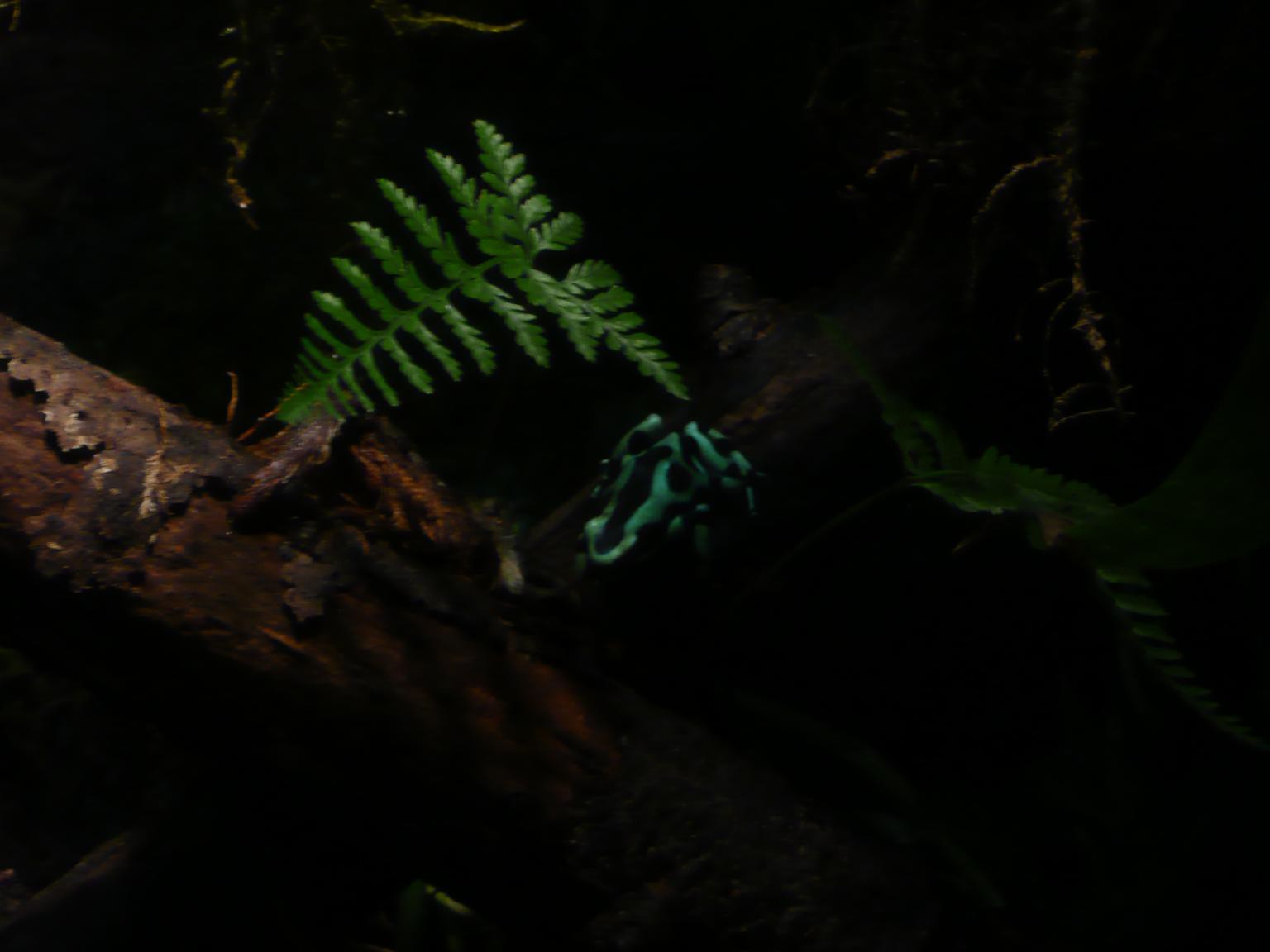In this very dark, nighttime photograph, a small poison dart frog with a striking green and black pattern is centrally positioned, facing the camera. The setting appears to be an outdoor forest environment. The frog rests on a piece of wood, which might be dead, surrounded by various natural elements. On the left side of the image, another piece of wood with a brown hue is visible, partially illuminated. Above the frog, there’s a fern or leafy plant adding to the greenery. The overall image is dominated by shades of black, green, brown, white, and gray, with no text present.